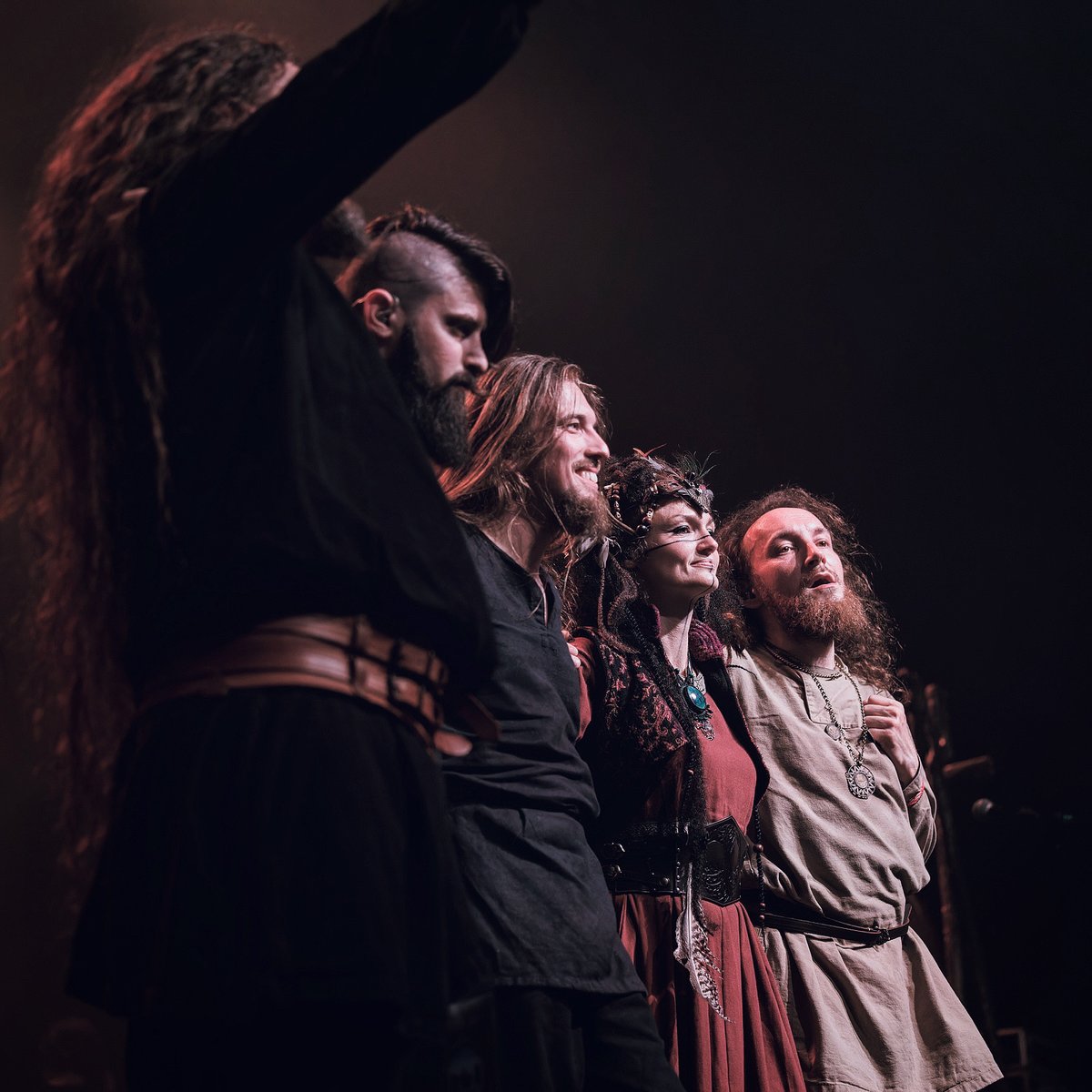The image depicts a left-side view of five individuals standing on a stage against a black background, arranged in a slightly outward curved line and looking to the right. They appear to be performers, possibly actors or singers, dressed in medieval or classical-style garments. On the far left is a woman with long dark, curly hair, wearing a black dress cinched with a brown leather belt, her raised arm obscuring her face. Next to her is a man with a black beard, mustache, and mohawk, dressed in dark clothing. The third person is a man with long, dirty blonde, streaky hair, a scruffy beard, and mustache, who is grinning, also dressed in black. The fourth person is a woman in a maroon dress, adorned with a black vest, a black belt, and a noticeable headdress, with a large blue stone necklace. Finally, on the far right is a man with dark curly hair and a beard, wearing a beige tunic with a black belt and a silver necklace. Some of the individuals appear to be either singing or smiling, adding a lively atmosphere to the scene.